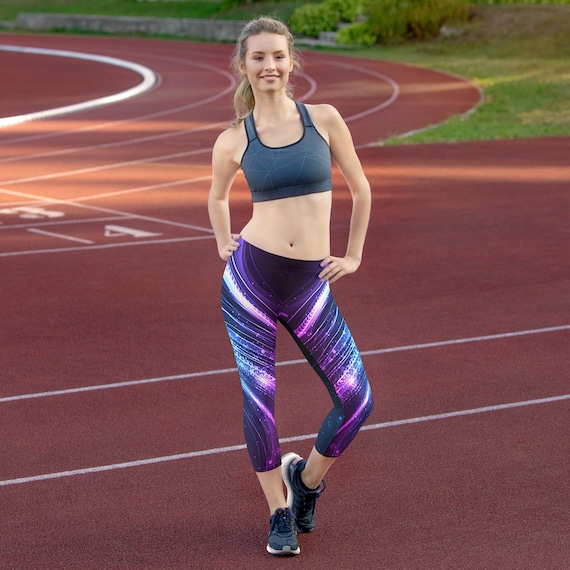This detailed photograph captures a young woman in her early 20s posing confidently on a traditional reddish-burgundy running track, marked with white lines and featuring visible track numbers. The track curves behind her, with grassy areas and bushes in the background. The woman stands with her hands on her hips, her left knee bent and her toe lightly touching the ground, giving a poised and somewhat playful appearance. She is dressed in vibrant, purple-striped three-quarter length yoga pants paired with dark-colored running shoes. Her gray sports bra reveals her toned stomach and complements the athletic ensemble. Her blonde, ash-brown hair is pulled back into a ponytail, and she's smiling lightly, with minimal makeup enhancing her natural features.